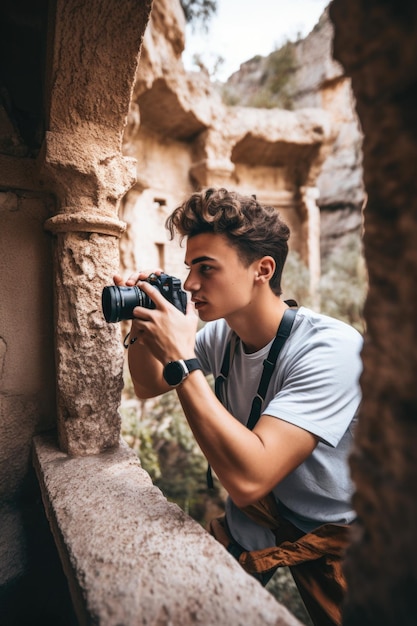This close-up angled photograph captures a young man, likely in his late teens or early 20s, standing amidst the ruins of an ancient building. The man, with his short, fashionably styled dark brown curly hair, wears a light blue t-shirt and has a brown shirt tied around his waist. On his right wrist, he sports a black watch. A camera with a long lens hangs from a strap around his neck, which he holds up to his eye as he peers through a rough, brown stone archway, likely reminiscent of Roman ruins with its curved formations. The scene suggests he is standing in the courtyard of these ruins, possibly at a ledge, taking a picture through the opening towards another part of the ancient structure. His chiseled features and poised stance add a youthful intensity to the photograph, set against the weathered backdrop of the historical architecture.